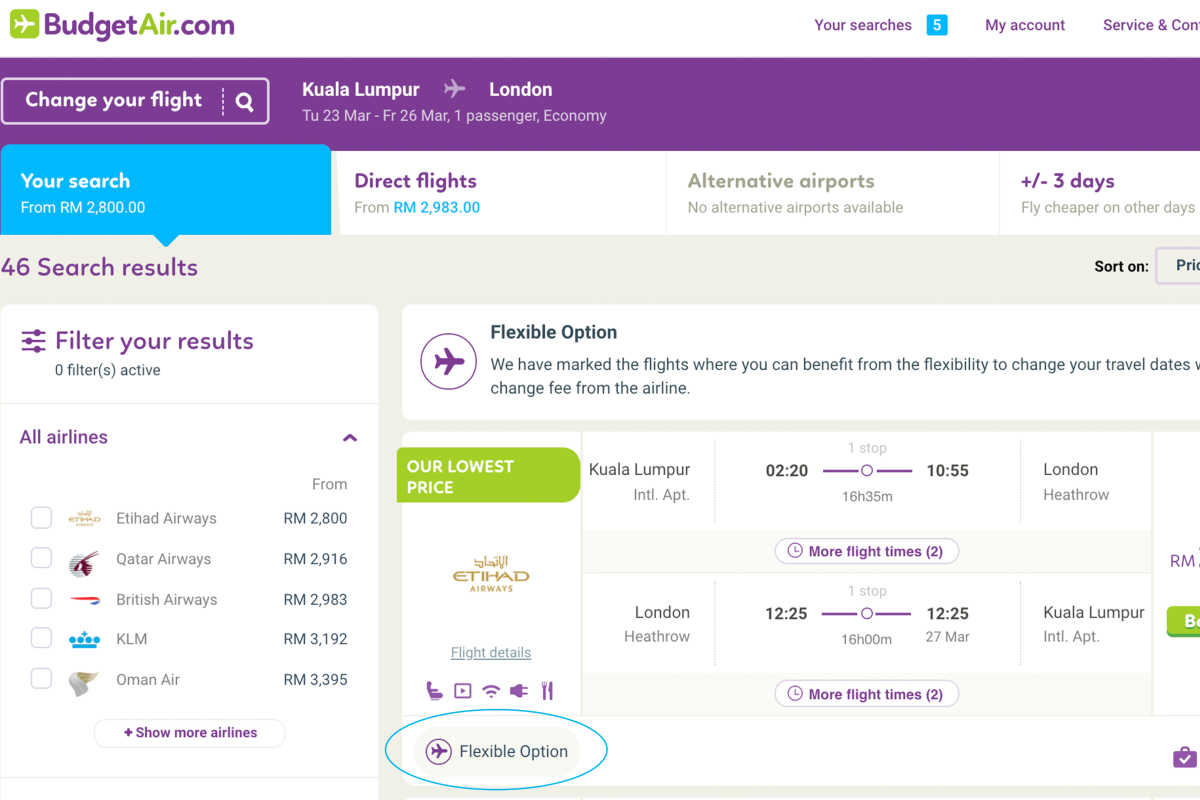The BudgetAir.com website features a clean, predominantly white design with eye-catching highlights of purple, lime green, and turquoise. The top left corner displays the BudgetAir.com logo, while the top right area houses navigation elements including 'Searches', which currently shows a count of five, 'My Account', and 'Services'. Beneath these elements is a distinct purple bar containing a search function labeled 'Choose Your Flight'.

The search interface showcases a sample flight from Kuala Lumpur to London, scheduled for Tuesday, March 23rd to Friday, March 26th, designed for one passenger traveling in economy class. A turquoise box indicates the starting price for this search at RM 2800, while a white bar beneath it lists direct flights starting from RM 2983. A dividing line splits this white bar, noting that no alternative airports are available. Another section within the same bar suggests considering travel dates within a range of plus or minus three days for potentially cheaper options.

Below the search details, a gray bar exhibits the total number of search results available, which in this scenario is 46. Users have the ability to sort these results via a drop-down menu, with 'Price' being the current selection. Additionally, the layout offers filtering options on the left-hand side, allowing users to narrow down their search results by their preferred airlines.